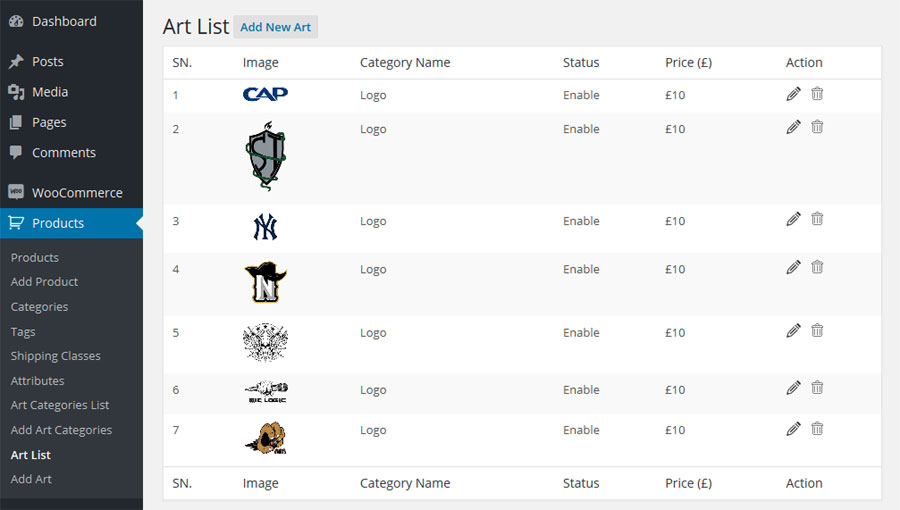In this detailed image description, imagine a screenshot depicting a WordPress admin dashboard interface with an off-white background and various listed items.

On the left side of the image, there is a black vertical sidebar with several menu items listed in white font. These items are each accompanied by small icons to their left. The listed entries include "Dashboard," "Posts," "Media," "Pages," "Comments," and "WooCommerce." Particularly noteworthy is the "Products" option, which stands out highlighted in a rectangular turquoise (or slightly darker blue) box and written in white font.

Beneath the "Products" section, a series of submenu items without icons appear. These are:

- Products
- Add Products
- Categories
- Tags
- Shipping Classes
- Attributes
- Art Categories
  - List
  - Add Art Categories
- Art List (bold white font)
- Add Art

Switching focus to the right part of the image, the central interface for managing products is displayed with an off-white background. At the top, a black bold title states "Art List." Directly below this title is a small horizontal rectangle with turquoise text that reads "Add New Art."

Within the off-white interface, a white rectangle is present, likely a table or grid containing categorized information. The table headers include "Categories," "Image," "Category Name," "Status," "Price," and "Action," each with a light horizontal line separating them.

Under “Categories,” labels denoted with capital letters such as "S. N." followed by a period are displayed, with a list of seven numbered items beneath it. The list is truncated at the bottom, ending with another “S. N.” suggesting more items are cut off.

Under the "Image" header, there are various logos including:
1. A navy blue word "CAP" in all caps.
2. A shield emblem.
3. The New York Yankees logo.
4. An "N" with a hat on it.

Some logos are too small to identify clearly.

For the "Category Name" column, all entries uniformly state "Logo."

Under "Status," every item is marked as "Enable."

The "Price" column shows a pound sign (£) followed by the number 10 (written as £10).

In the "Action" column, there are icons of pencils followed by trash can icons, indicating options to edit or delete each entry.

This detailed description encompasses the layout and specific content illustrated in the image, giving a clear visual of the WordPress admin dashboard interface for managing products.